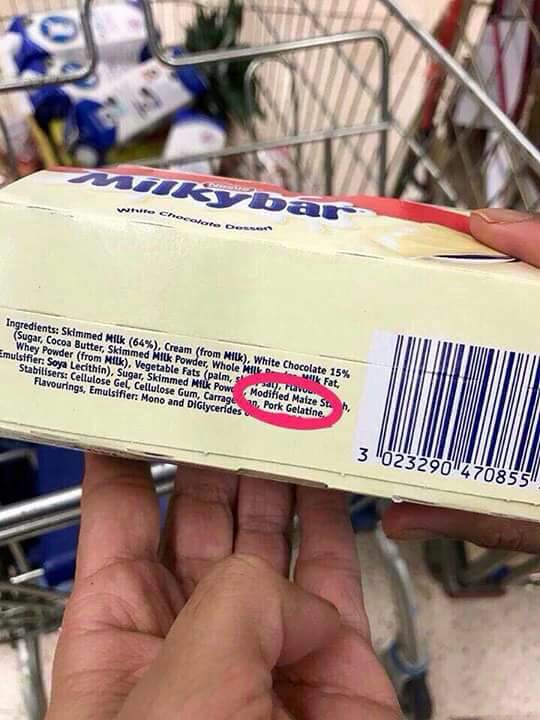In this photograph, a shopper is seen in a grocery store holding a beige box labeled "Milky Bar White Chocolate Dessert." The person holds the box with their left hand supporting it from the bottom and their right hand grasping it from the side, positioning it above a metal chrome shopping cart that features a blue baby seat. The shopper's cart contains various items. The focus of the image is on the bottom of the box, where the ingredient list and barcode are visible. Notably, a red circle highlights the mention of "Modified Maize" and "Pork Gelatin" among the ingredients. The box prominently lists ingredients such as 64% skim milk, 15% white chocolate, sugar, cocoa butter, various milk derivatives, vegetable fats, soy lecithin, and modified maize.